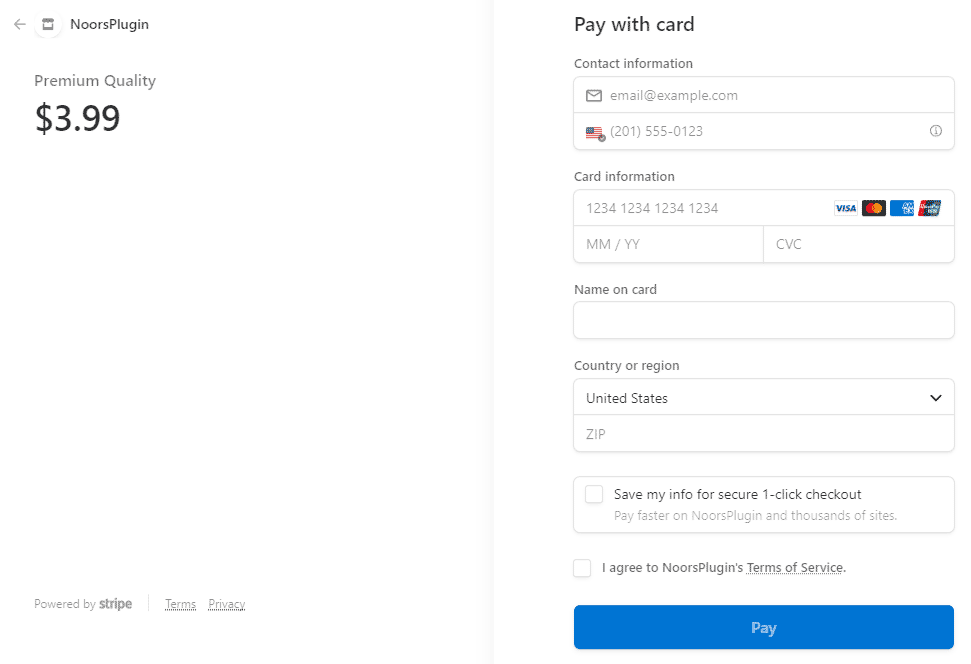The webpage features a streamlined payment interface divided horizontally into two sections. The left section displays minimal content, prominently highlighting the product being purchased: "Nor's Plugin" in small gray font at the upper left corner. Below, also in gray, is the tagline "Premium Quality." The price, $3.99, stands out in bold black font. The remainder of this section is blank.

In contrast, the right section is more detailed, beginning with a conspicuous "Pay With Card" header. Directly beneath is the "Contact Information" section, featuring fields for entering an email address and a phone number. Following this is the "Card Information" section, which includes a field for card details with an example number (1234 1234 1234 1234) displayed. Accompanying this are icons for various credit card types. Below, fields for the card's expiration date and CVC code are provided, along with a "Name on Card" field.

Further down, there's a "Country or Region" dropdown menu, preset to the United States, and a field for entering a zip code labeled "Zip." At the bottom, there's an option to save payment information for future purchases, explained in a small rectangular area with a checkbox for "Save My Info for Secure One-Click Checkout. Pay Faster on Nor's Plugin and Thousands of Sites." Beside it, another checkbox allows the buyer to agree to Nor's Plugin's terms of service. Finally, a prominent blue "Pay" button completes the form at the bottom of the page.